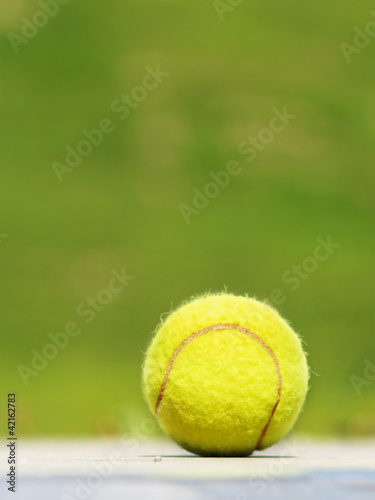The image features a bright, lemon-yellow tennis ball set against a green upper background and a light beige or cream lower surface. The focus is on the tennis ball, prominently displaying its brownish curved seam running from the top to the bottom. The surfaces in the background are slightly blurred, emphasizing the detail of the tennis ball, including its fuzzy texture. A soft shadow is cast beneath the ball due to overhead lighting. The entire image is overlaid with Adobe Stock watermarks, and the bottom left corner is marked with "Adobe Stock 42162783," indicating its licensed stock number.